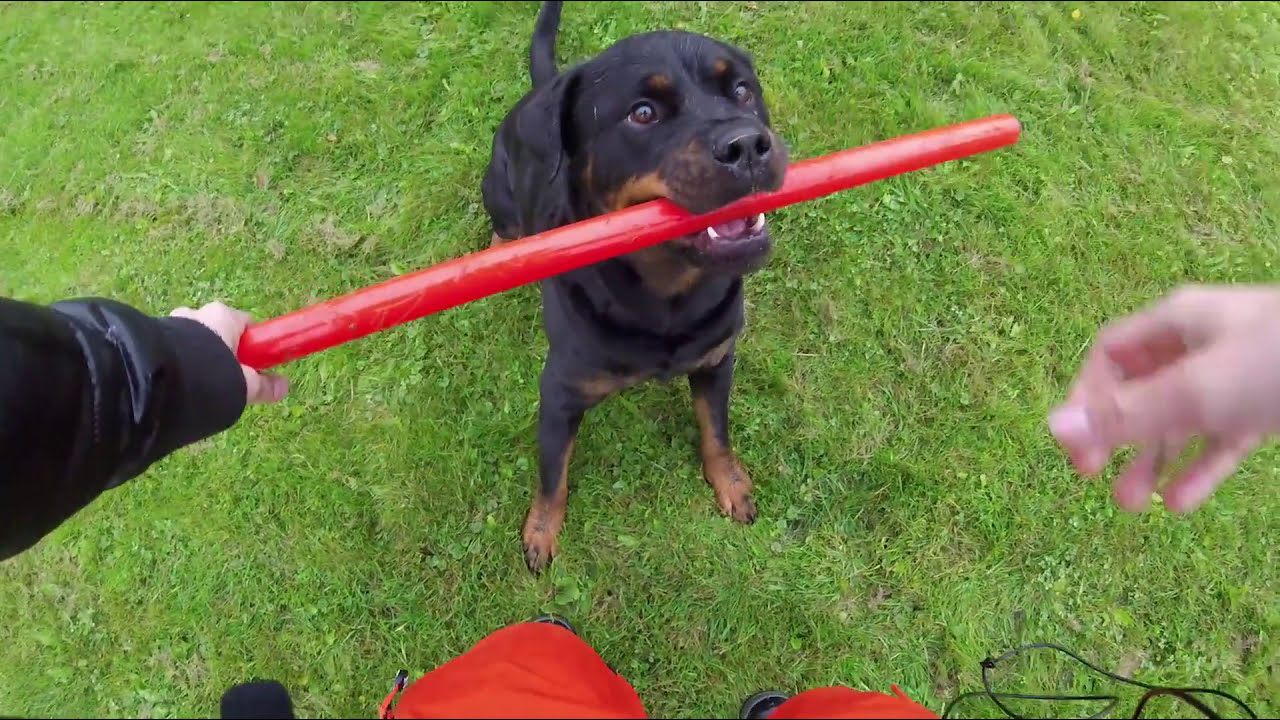In this vibrant daytime photograph, a Rottweiler with a predominantly black coat and distinctive brown markings around its mouth and feet engages playfully with its owner on a freshly mowed grassy lawn, likely in a park. The image, taken from a GoPro perspective, shows the dog seated and looking up, gripping one end of a long, red, plastic stick with its mouth, while the person holds the other end in their left hand. The person, shown from the waist down, is wearing a black jacket, red pants or shorts, and black shoes. Their other hand, slightly motion-blurred, appears on the right side of the image, emphasizing the dynamic interaction and playful tug-of-war between the two. The light conditions and the partly cloudy sky suggest that the picture was taken during the daytime.